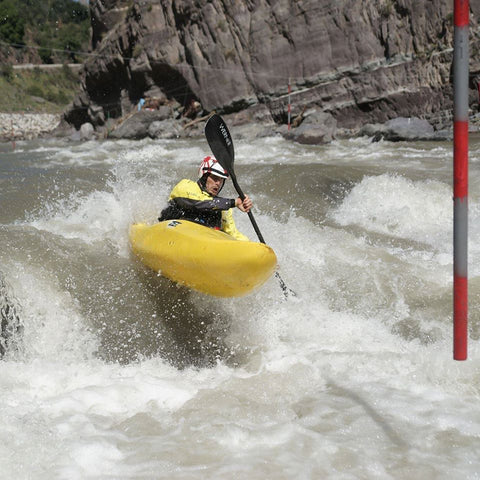The photograph captures an intense action shot of a man in a yellow kayak navigating through tumultuous whitewater rapids. Dressed in a yellow life jacket over a black long-sleeved shirt and a distinctive white helmet with red designs, he maneuvers his black paddle to steer through the foamy, brown waters. The yellow kayak, partially lifted above the wild current, emphasizes the sheer force of the rapids. The backdrop reveals rugged cliff faces and eroded mountain terrain that frame the river, with rocks, trees, and brush lining the sides. A striped red and gray pole is visible in the water, adding an extra element to the scene. The image's composition and the man's focused expression, facing towards the camera, make for a compelling depiction of the thrill and challenge of whitewater kayaking.